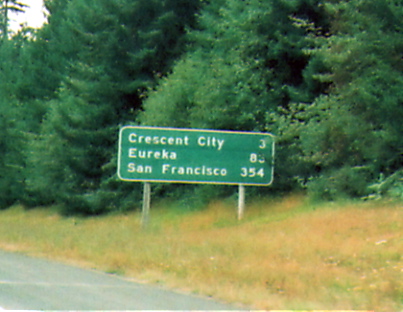The image depicts a green mileage highway sign mounted on two grey metal poles. The sign, with a white outline and white letters, lists the distances to three cities: Crescent City (3 miles), Eureka (83 miles, partially obscured by a tree branch), and San Francisco (354 miles). Behind the sign is a dense forest of tall, green trees. In the foreground, there is a mix of yellow, green, and brown grass, with a grey road visible on the bottom left. The sky peeks through in the left-hand top corner, adding a touch of white to the scene.